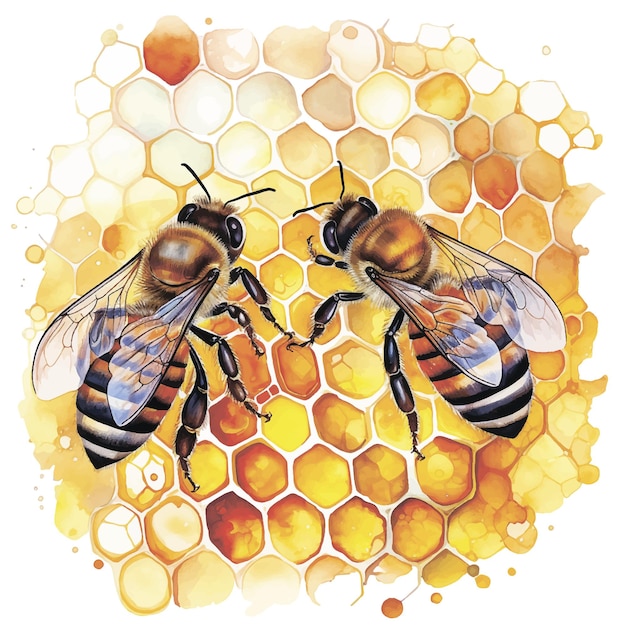This detailed watercolor illustration depicts two large honey bees with yellow and black striped, hairy bodies, and prominent antennas. The bees, with their intricately detailed wings, are positioned diagonally on a vibrant honeycomb composed of hexagonal cells filled with golden honey. The bees' heads are angled towards each other, almost touching, adding a dynamic element to the composition. The honeycomb structure, predominantly yellow, gradually fades into white towards the edges of the image, highlighting the bees and their environment. The overall color palette includes shades of black, brown, gold, orange, yellow, beige, tan, and white, contributing to the lifelike and vivid portrayal of the scene. The piece, either drawn, painted, or digitally created, masterfully captures the texture and intricate details of the bees and their honeycomb backdrop.